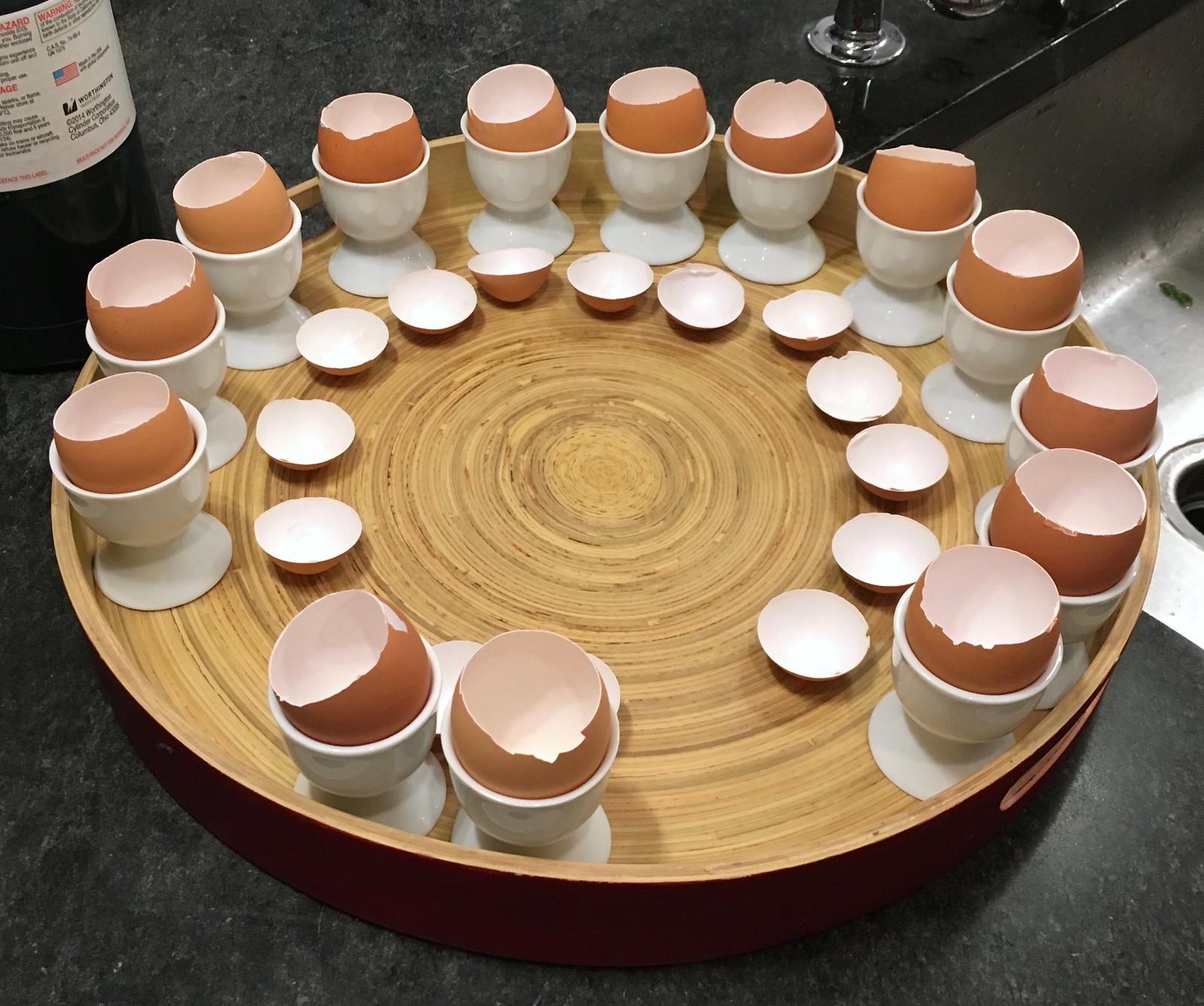This photo depicts a round wooden serving platter, its outer edge tinged with a reddish hue, sitting on what looks like a kitchen or restaurant counter, likely granite. The platter is adorned with approximately 16 small white ceramic cups, each containing a brown egg with its top meticulously removed. The cut-off tops of the eggshells are placed with the inside facing up, arranged outside the cups to form a fairly concentric circle. However, two gaps in the circle can be observed at about five o’clock and seven o’clock. The setting includes a glimpse of a sink to the left and a bottle with a white label and an American flag at the top right, possibly hinting at an alcoholic beverage.